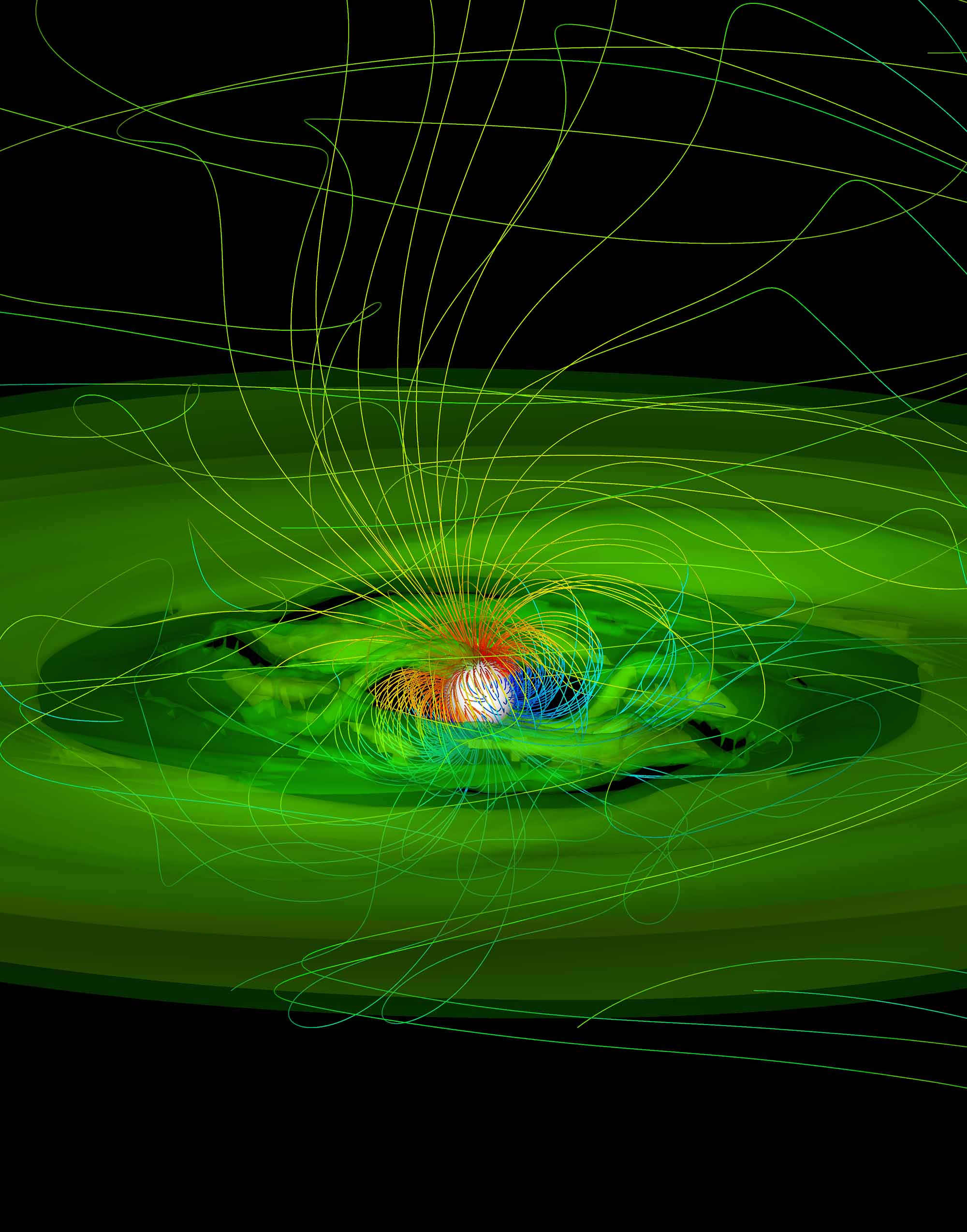The image depicts a surreal, cosmic scene with a mysterious central structure. At the core, a bright white sphere radiates an array of vibrant colors, including reds, oranges, blues, and yellows. Surrounding this central sphere, a swirling nebula of neon green gas forms a circular cloud-like structure. From the heart of this nebula, numerous yellow filaments or wires emanate, extending outwards in all directions, creating a pattern reminiscent of magnetic field lines. These filaments become less concentrated as they spread out, yet some continue to swirl and twist all the way to the edges of the image, which is set against a deep black background. The overall effect is that of a dynamic, luminous aura with a chaotic yet mesmerizing arrangement of colors and lines, evoking images of a digital or cosmic phenomenon.